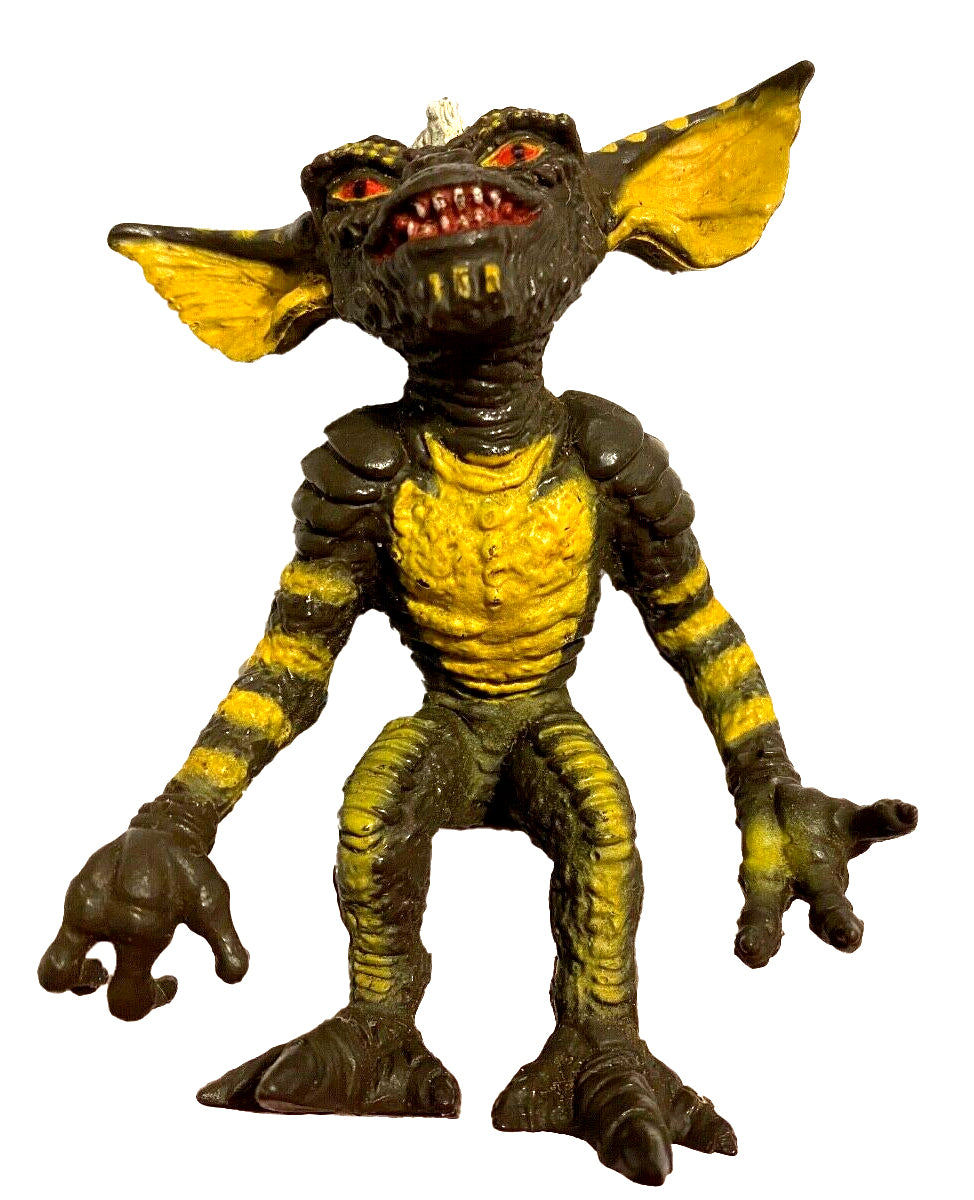The image features a detailed, menacing toy from the Gremlins franchise against a white background. The creature, resembling a fantasy goblin, has predominantly black or dark green skin with distinctive yellow patterns. Its solid yellow torso contrasts with the yellow stripes on its long arms and the fronts of its legs. The creature's face is particularly striking, with large bat-like ears that have yellow lining and additional yellow dots on the upper ears and where eyebrows would be. Its eyes are narrow, with red backgrounds and black, slit pupils akin to a reptile's, giving it a penetrating gaze. The mouth is wide open, showcasing pointed white teeth set in a red-painted mouth, with three characteristic yellow lines on its chin.

A small horn protrudes from its forehead, adding to its formidable appearance. The monster has heavily ridged shoulders that look like layered armor or pauldrons. Its arms are exceptionally long, extending down to its knees, each ending in three-fingered hands with long nails. Its feet are flat, with three clawed toes each, similar to a dinosaur’s, and they appear somewhat webbed. The overall look is completed with a scaled texture covering its body and an expression that implies it is looking slightly upwards, adding to its eerie impression.